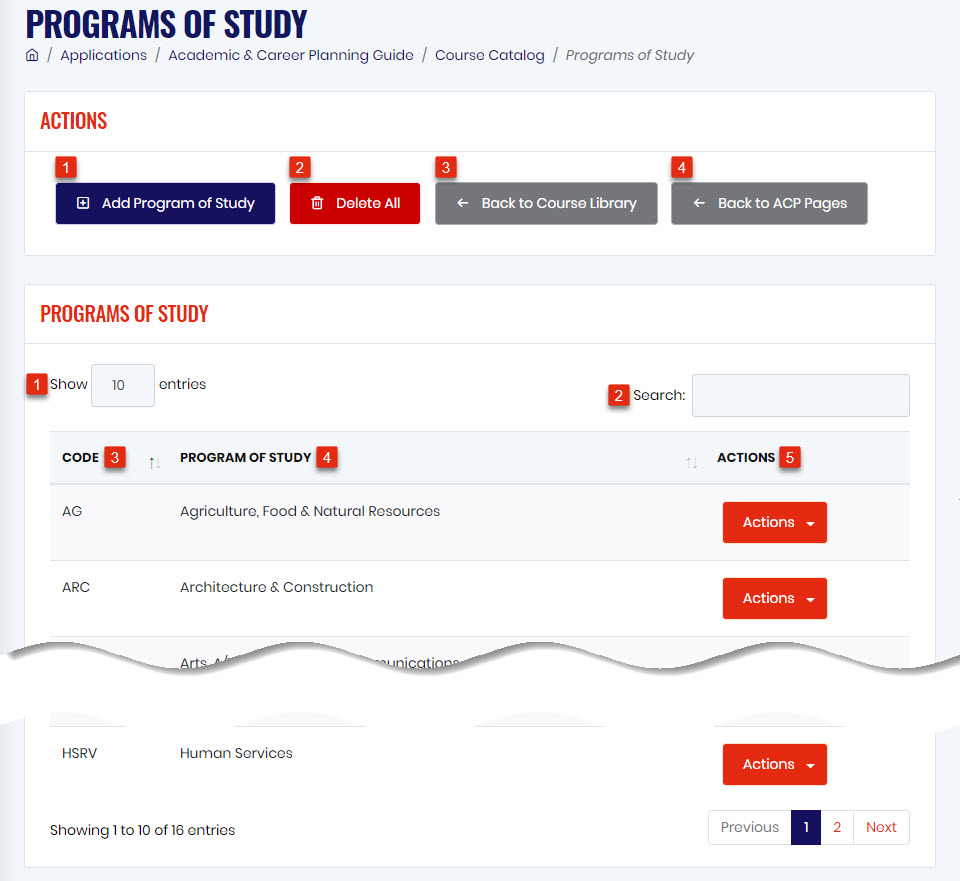The image portrays a laptop screen displaying a web interface for an academic and career planning guide and course catalog. The title "Programs of Studies" is prominently featured in dark blue text at the top of the screen. To the left of the title is a home icon, and to the right, there is a navigation path indicating the sections "applications" and "academic and career planning guide."

The background of the screen is a light blue or gray, with several functional boxes outlined against this backdrop. At the top, there are several action buttons. On the top left, a red "Actions" button is visible. Below that, there's a dark blue bar labeled "Add Program of Study," and next to it, a red bar labeled "Delete All." Further to the right, a gray bar with a back arrow indicates "Back to the Course Library," and another gray bar mentions "Back to ACP Pages." Additionally, there's a sequence marker in a red box noting "1, 2, 3, 4," which likely represents steps within the interface.

Below this top section, the screen splits into different sections. The label "Programs of Study" appears again, noting the ability to "show 10 entries" on the left and a search bar on the right. The table beneath this header lists codes and programs of study with corresponding action buttons on the right side for each entry. The codes include AG (Agriculture, Food, and Natural Resources), ARC (Agriculture, Construction), and HSRV (Human Services). These entries are separated by visual breaks, separating sections distinctly.

Lastly, at the bottom left of the screen, there is pagination information indicating "showing 1 to 10 of 16 entries," providing the user with navigational context for the data displayed.